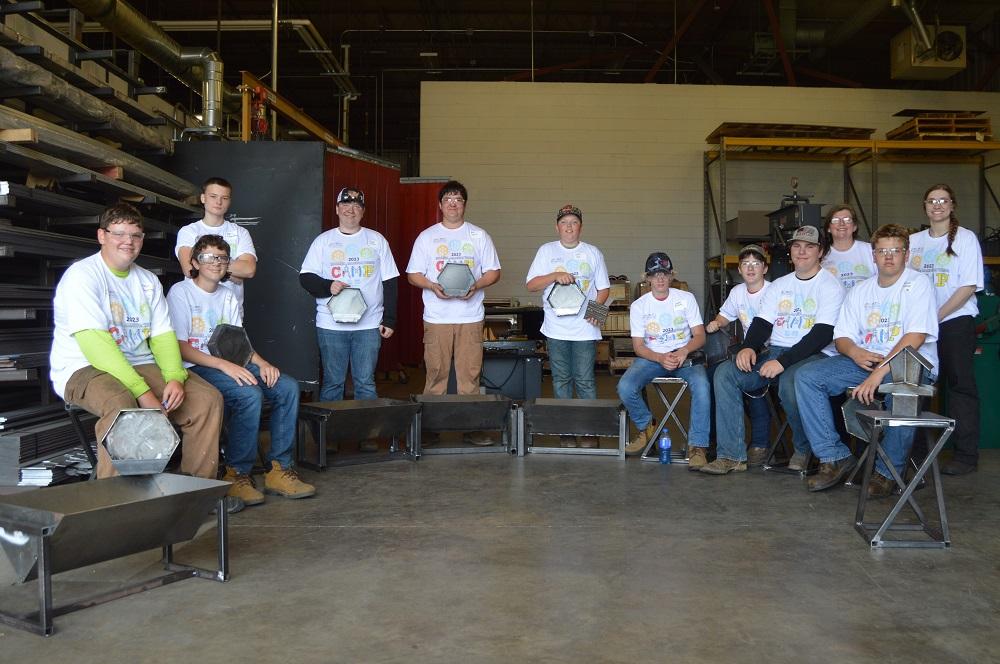This photograph captures a group of 12 individuals in a semicircle inside what appears to be a metal workshop or production facility, characterized by its cement flooring and stacks of supplies, possibly sheets of metal or lumber, in the background. The group consists of a diverse range of people, including both males and females, and varies in age from teenagers to possibly young adults. They are all wearing the same branded white t-shirt featuring bright, rainbow-colored letters, blue jeans, and boots, with some donning safety glasses while others do not.

Notably, they are holding various metal creations they have crafted, including hexagonal shapes and a metal side table with a birdhouse on top. Their expressions vary, with some beaming at the camera and others looking less enthused. The overall setting, coupled with the attire and creations, suggests that they might be participants in a welding class or workshop, celebrating a moment of achievement possibly signified by the awards some of them are holding.